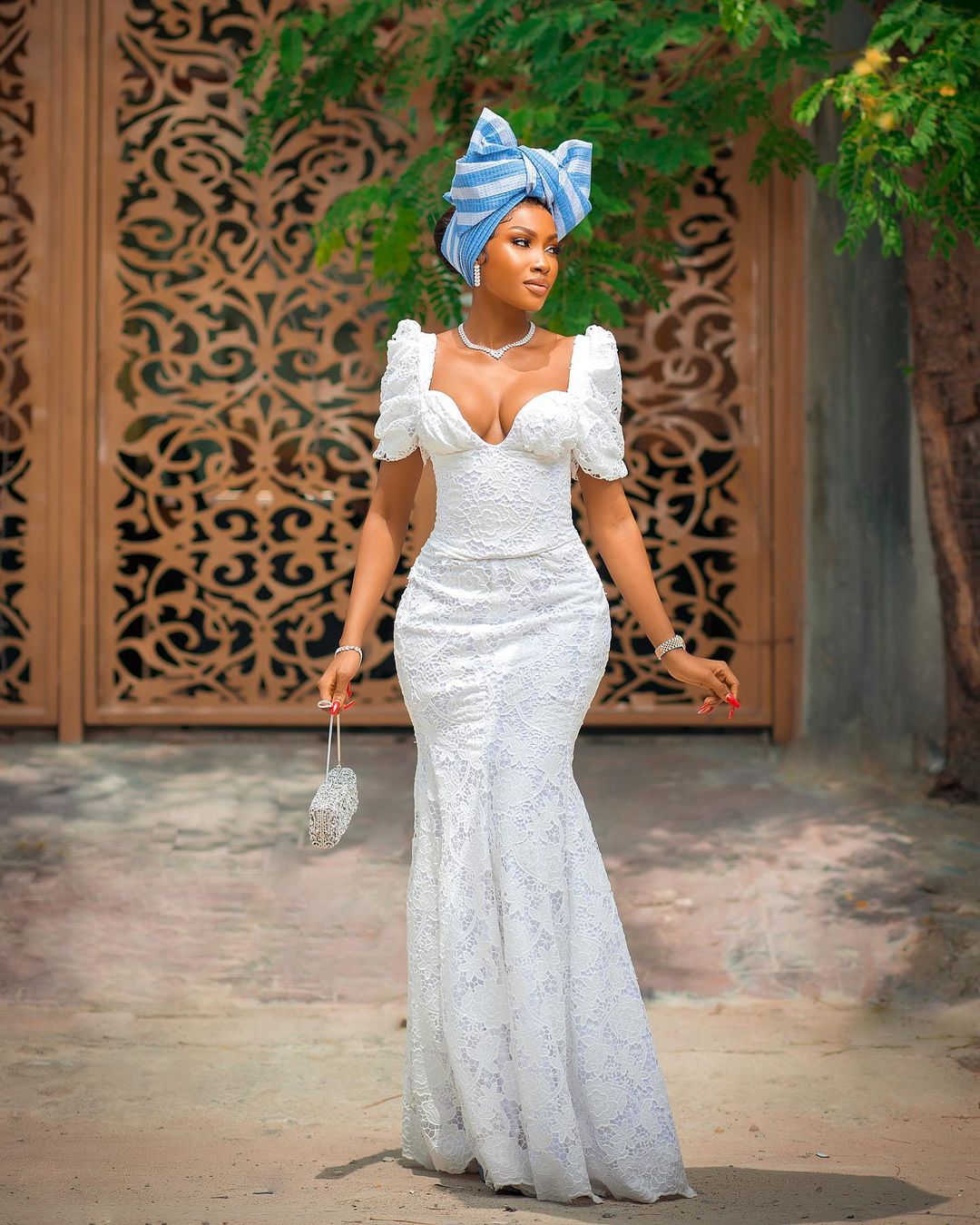In this captivating outdoor portrait, a medium complexion African American woman is elegantly posing while looking off to the left, allowing for a clear view of the right side of her face. Her black hair is gathered into a bun, partially obscured by a stylish head wrap featuring medium blue and white stripes, adorned with a prominent bow at the front. She is resplendent in a floor-length, form-fitting white lace dress that cinches at the waist and flares out in a mermaid style. The dress features elbow-length puffed sleeves and a scooped neckline that reveals a hint of her décolleté. 

Her makeup is subtly done with nude tones on her lips and eyes, complementing her natural beauty. Her ensemble is accessorized with a sparkling diamond choker necklace, silver earrings, a sparkling wristwatch on her left wrist, and a silver bracelet on her right wrist. She further accentuates her look with red nails and a glitzy clutch adorned with crystals.

The background reveals a rust-colored, filigree-like metal gate and a tree, adding a natural element to the scene. The woman stands on a tan surface, possibly concrete, under the bright daylight, not engaging directly with the camera, which adds a sense of candidness to the photograph. The entire setup and her poised demeanor exude grace and sophistication.